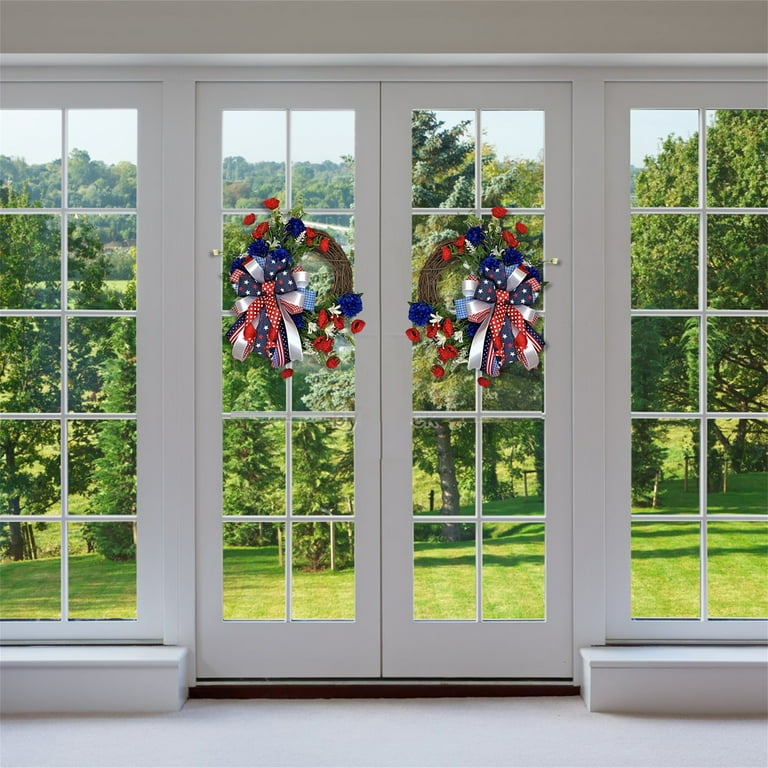The image captures a bright, daytime scene from inside a house, showcasing a pair of full-length glass double doors adorned with festive wreaths. Each door has ten glass panes and is framed in crisp white molding. Flanking the doors on either side are additional matching windows, similarly detailed with white, painted woodwork. Hanging on both doors are red, white, and blue wreaths, complete with patriotic ribbons, indicating 4th of July decorations. Through the glass panes, one can see a lush green lawn stretching out into a large backyard, bordered by trees and hinting at a distant fence line. The scene evokes a sense of celebration and openness, with the vibrant greenery visible outside contrasting with the intricate, clean lines of the white doors and windows.